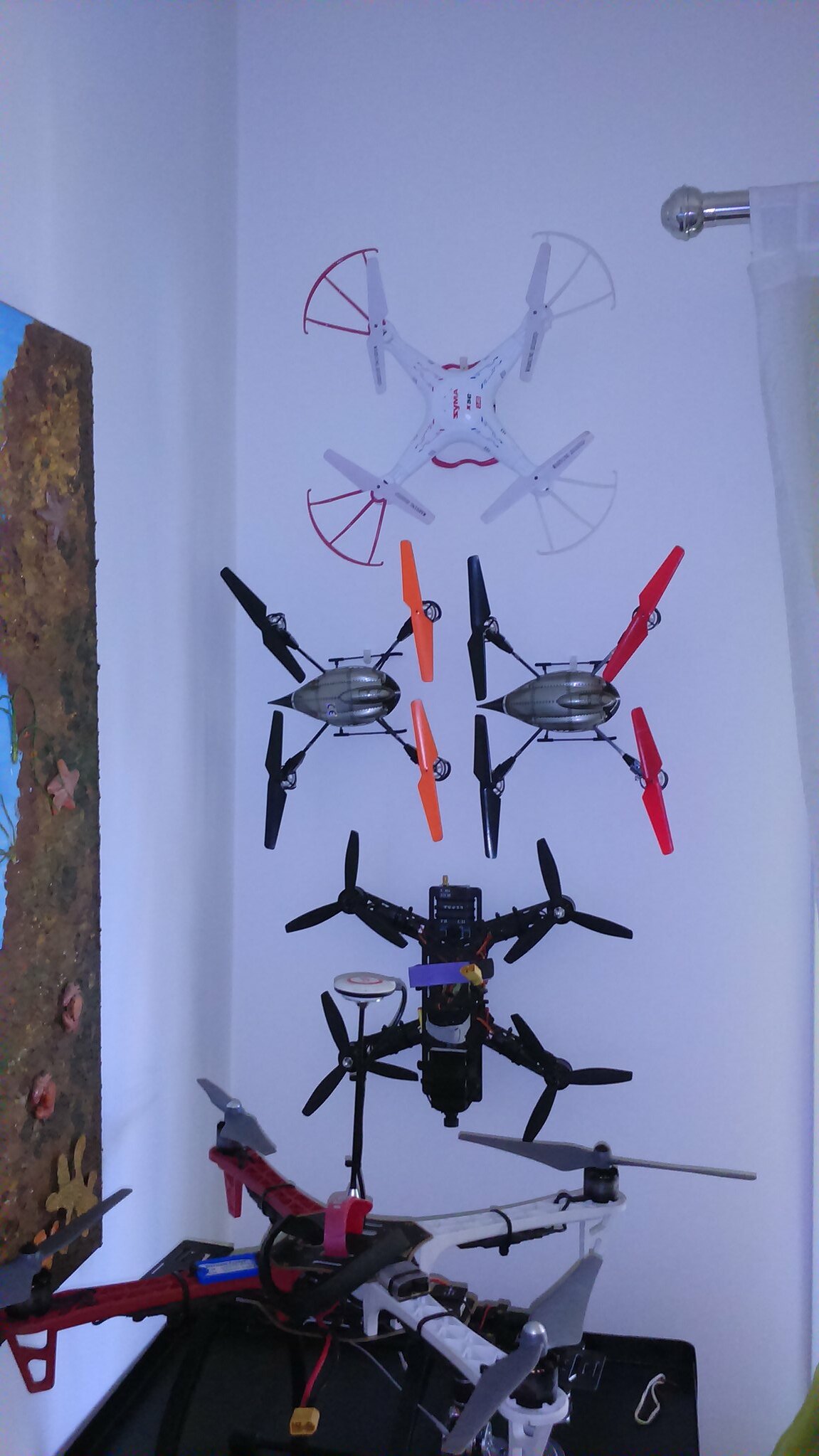In a room with white walls and a sheer white curtain partially visible on a curtain rod at the top, there is a black dresser or chest adorned with a white rubber band. On the dresser sits a white and red model drone with gray propellers. Above it, several drones appear to be hovering at different levels against the wall. The largest white drone has an X shape with red propellers on the left and white propellers on the right. Two medium-sized drones feature black and orange propellers, with one sporting red and black colors. At the bottom, a smaller drone has black propellers on all four sides. Additionally, a dark brown and tan corkboard with blue and brown elements is on the left wall. The arrangement and suspension of the drones create a seemingly floating display, making it appear as if they are in flight.